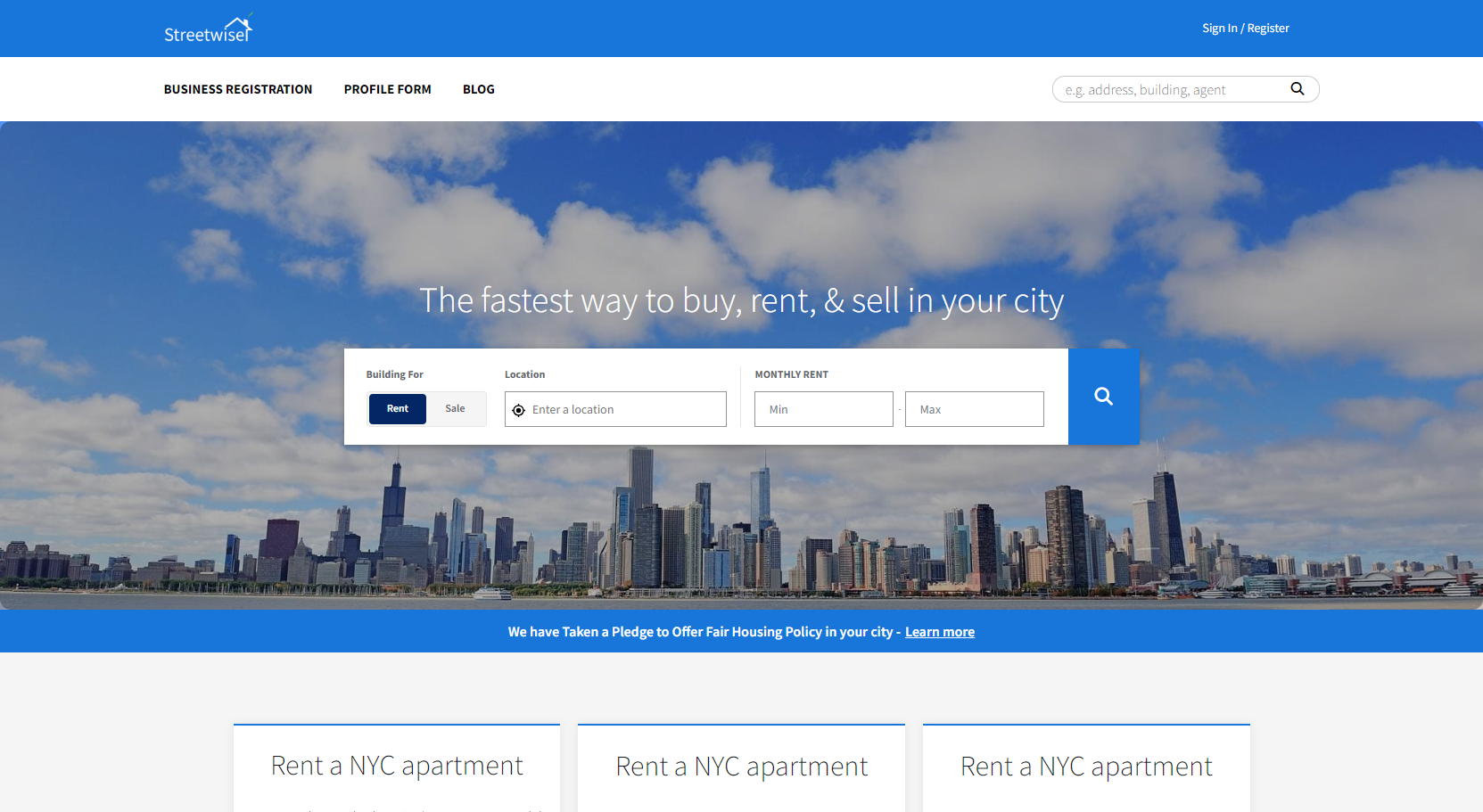The image displays the home page of a website named "Streetwise." In the upper left corner, a house icon serves as the logo, situated above the word "Streetwise." To the far right at the top, there are options for users to sign in or register.

Beneath the "Streetwise" header on the left side, three categories are listed in black text: "Business Registration," "Profile Form," and "Blog." On the far right is a search bar with a gray placeholder text that reads "e.g., address, building, agent," accompanied by a black magnifying glass icon on its right side.

Dominating the central portion of the page, a bold statement reads, "The fastest way to buy, rent, and sell in your city." Below this, a framed section features text fields and buttons to assist users in their search. The first box prompts for "Building" followed by options to "Sell" and "Buy." Adjacent to this, another box requires a "Location," and next to it, fields for "Monthly Rent" display "Min" and "Max" labels. A white magnifying glass icon is positioned to the right of these fields for initiating the search.

The background of the page presents a city landscape, featuring high-rise buildings against a bright blue sky dotted with white clouds. Additional elements of the scenery include a beach area, adding a scenic touch to the urban backdrop.